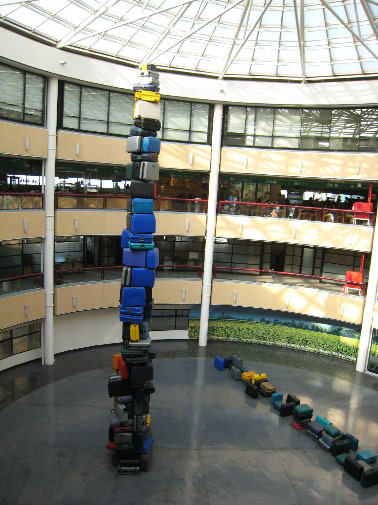The image features the interior of a circular, four-story building with a glass dome ceiling supported by visible metal struts and glass panels. The perspective is from the third floor, looking into an open courtyard at the center of the structure. The courtyard floor is made of dark stone or concrete and is shiny and reflective. The space features an intriguing installation of luggage in vivid colors like turquoise, blue, yellow, and red. A line of suitcases stretches from the right bottom corner to the center of the image, while another vertical stack of luggage, resembling a Jenga tower, ascends past the fourth floor, nearly reaching the glass dome. Each floor encircles the courtyard, with beige balconies and red guardrails complementing the modern design. Sculptures are visible within the courtyard, adding to the artistic ambiance of the space. The surrounding floors house various rooms or offices, partially visible in the background.